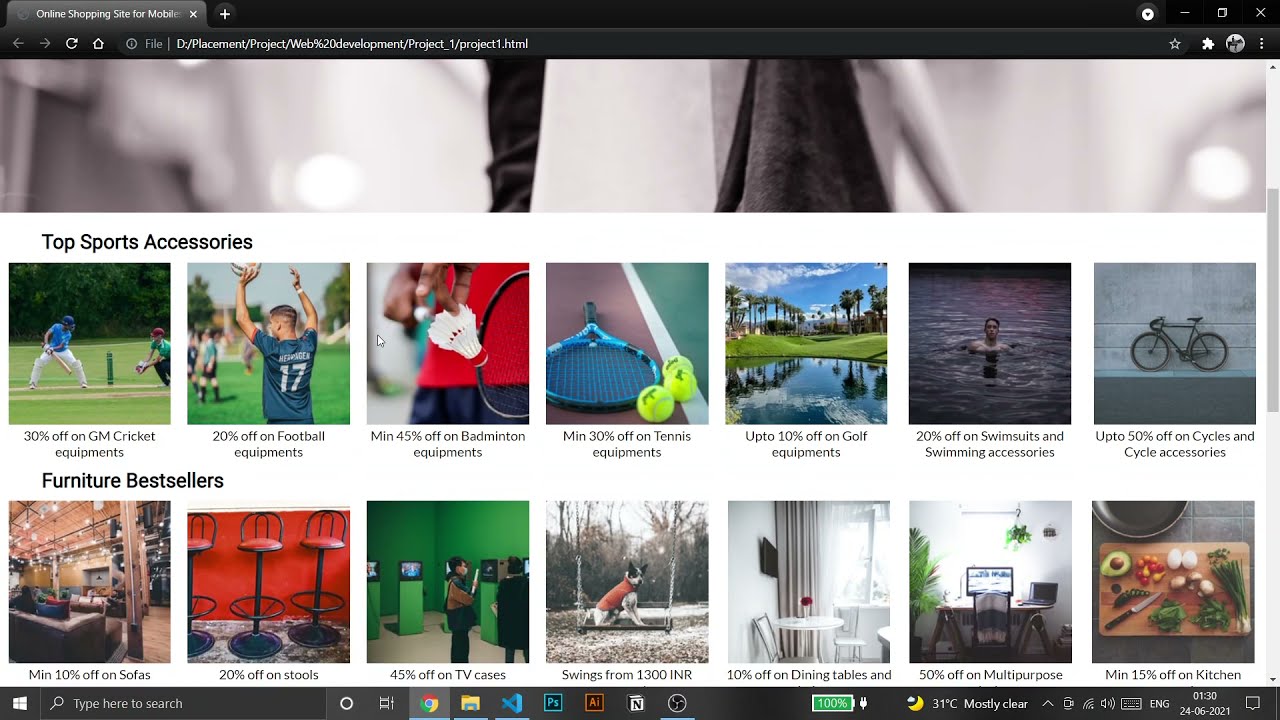The image depicts the interface of an online shopping site for mobile devices. 

At the top, there is a dark grey tab with white text displaying "Online Shopping Site for Mobiles". Next to it is a black circle featuring a white plus sign, which appears to be for adding another tab. Moving across the top bar, there are various symbols: a black circle, a white circle, a black triangle, a white dash, an outlined white box, and a white 'X' signifying different interface elements.

Beneath this top bar, on the left side, are icons including a left-pointing arrow, a right-pointing arrow, a circular refresh button, and a house icon indicating the home button. There is also a grey browser box displaying the file path: "file:///D:/placements/projects/web%20developments/project_one/project_one.html".

Further, symbols such as an outlined white star, a white puzzle piece, and a black circle are present, though not all details are clear.

The main body of the page has a white background with black text listing offers and categories. It advertises:
- 30% off on GM cricket equipment,
- 20% off on football equipment,
- Minimum 45% off on badminton equipment,
- Minimum 30% off on tennis equipment,
- Up to 10% off on golf equipment,
- 20% off on swimsuits and swim accessories,
- Up to 50% off on cycling and cycling accessories, with a feature on furniture bestsellers.

This detailed description captures the layout and features visible in the screenshot of the online shopping site.